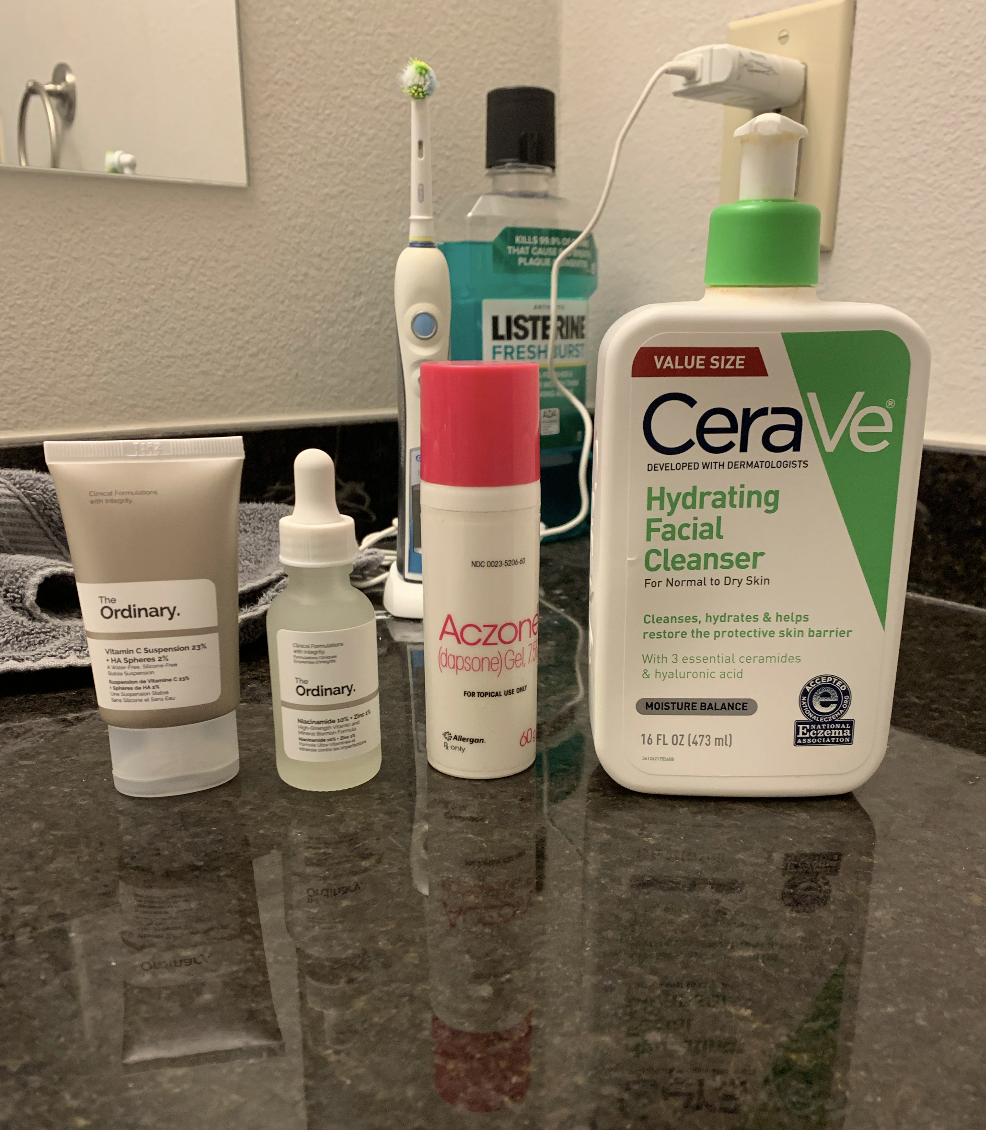The image captures a meticulously organized bathroom countertop. Central to the display are several bottles, each neatly lined up in a row. The lineup starts with a white bottle of CeraVe facial cleanser, distinguished by its green and white lid. Beside the cleanser is a white bottle of Xone gel, easily identifiable by its red top. Adjacent is a clear dropper bottle, complete with a white dropper top and label. On the far left, there is a squeeze bottle containing a beige substance, accented with a white label and a clear cap.

The countertop itself is strikingly black, featuring a highly glossy and reflective surface that contrasts with the arrangement of bottles. In the backdrop, a blue bottle of Listerine with a black lid stands behind the foregrounded items, adding a pop of color. An electric toothbrush with a green head and a blue button is plugged into the wall, ready for use. A gray towel lies folded behind the bottles, adding a touch of softness to the scene. The wall behind the countertop is painted white, providing a clean and minimalist setting. To the left, a mirror is mounted on the wall, reflecting the organized space and amplifying the room’s brightness.